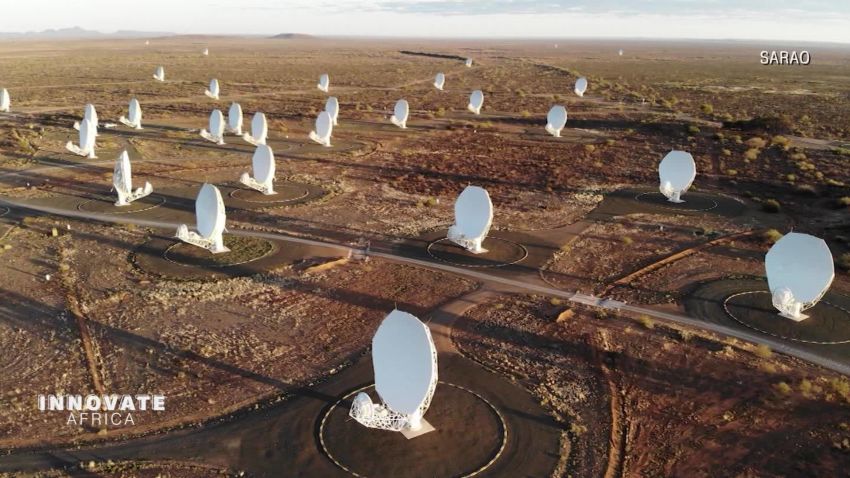The image depicts a sprawling, open field featuring numerous bright white satellite dishes, likely located in Africa as suggested by the text "Innovate Africa" in white block letters and "SARAO" in the top right corner. Captured from an aerial perspective, possibly by a drone, the field below is a mix of earthy tones—red and yellow hues—with each satellite dish encircled by a lined fence. The dishes, which appear hexagonal or octagonal, are positioned in a circular arrangement throughout the field, spaced far apart from each other for optimal placement. A road stretches across the image from the center right side to the bottom left, facilitating vehicular access. In the background, a couple of hills can be faintly seen on the top left corner, adding to the vastness of the landscape.